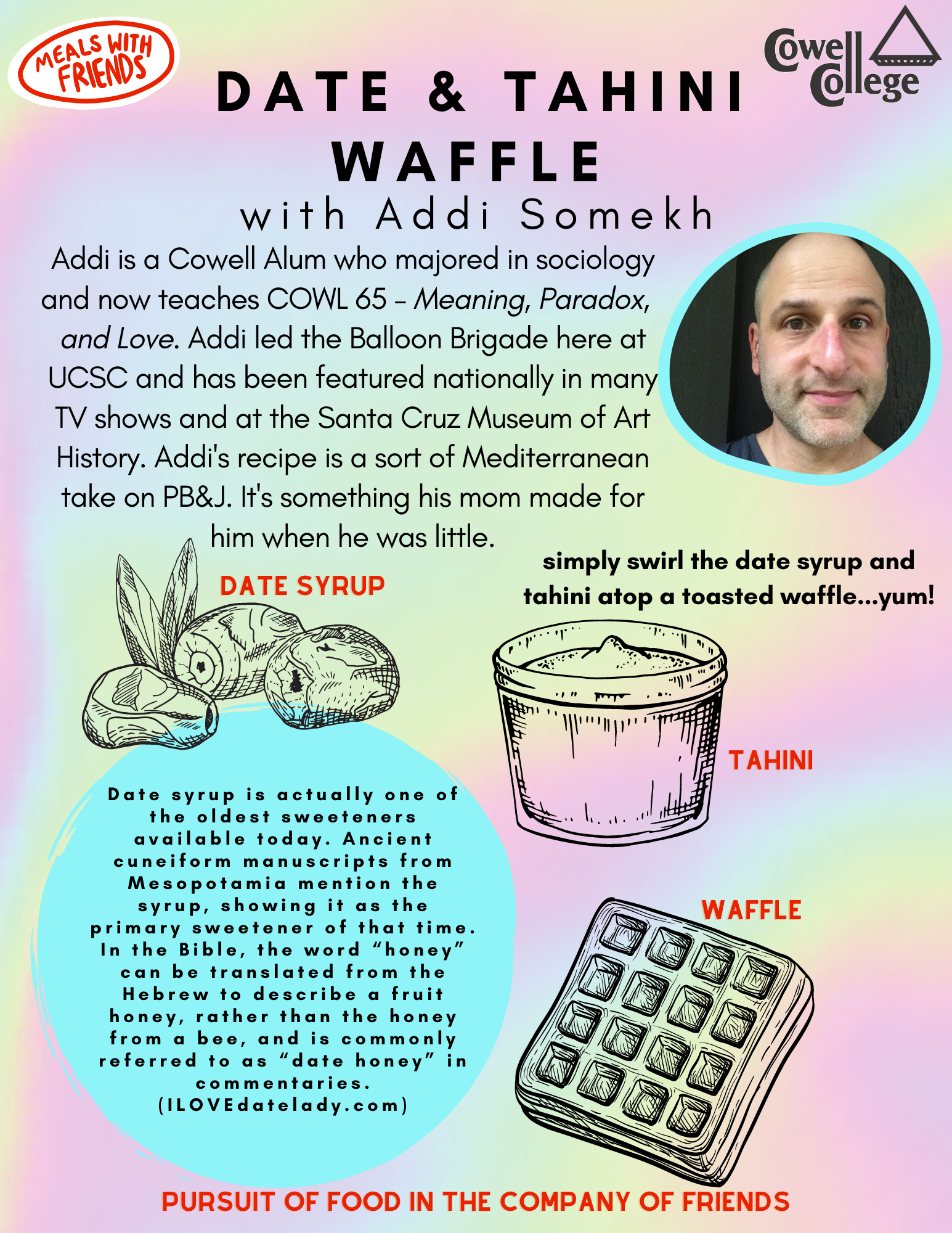The poster showcases a recipe for Date and Tahini Waffle, set against a watercolor-like pink and blue background. In the top left corner, a red-outlined white oval displays "Meals with Friends" in red. The top right corner features "Cowell College" in black with a triangle logo. Centrally located is the title "Date and Tahini Waffle with Addy Somek," followed by a biography of Addy Somek – an older, light-skinned man whose photo appears to the right in a blue-outlined circle. A detailed description of date syrup is placed at the bottom within a large blue circle. Instructions are clear: "Simply swirl the date syrup and tahini on top of a toasted waffle." The poster also includes clipart images of a waffle, tahini, and dates. Concluding the design, the phrase "Pursuit of Food in the Company of Friends" is prominently displayed in red at the bottom.